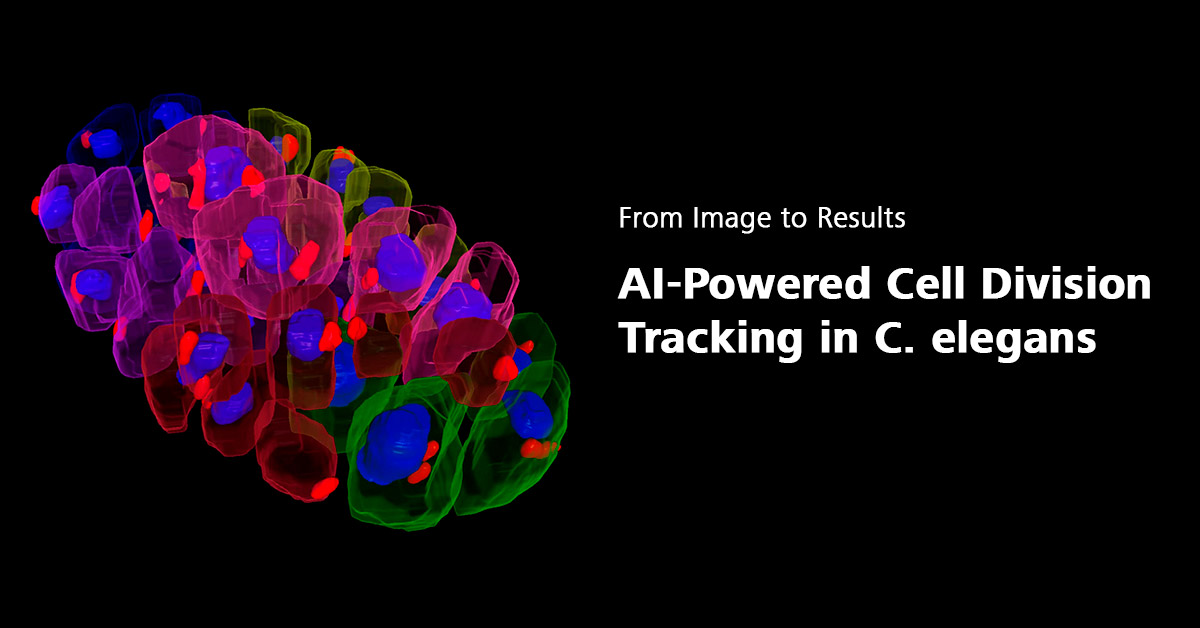The image features a black background with white block lettering that reads, "From Image to Results, AI-powered cell division tracking in C. elegans." On the left side of the image is a vibrant and colorful illustration resembling a 3D model of cells in division. The illustration is composed of various bright, neon colors including pink, purple, blue, green, red, and orange. The cells appear as amorphous blobs, with green circles containing blue and red inner circles and smaller red spots scattered throughout. The overall shape of the illustration is reminiscent of an ornate coral reef or a pine cone, creating a visually striking and intricate design. The detailed and vibrant depiction emphasizes the advanced technology of AI in tracking cell division in C. elegans.